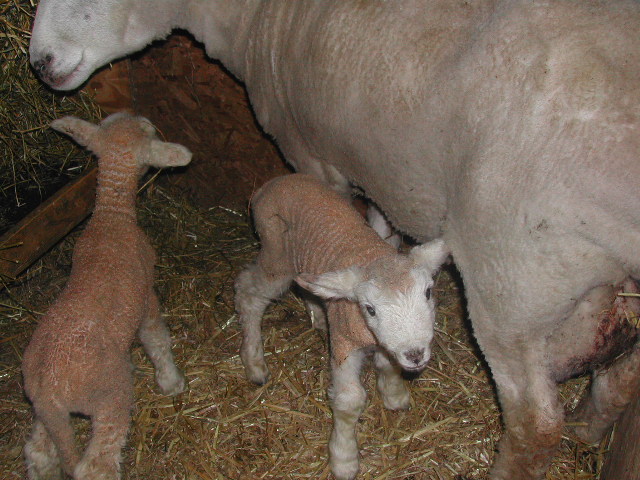This photograph depicts a farm scene with a recently sheared mother sheep and her two very young lambs, standing on a bed of straw. The mother sheep, whose mostly white body curves around the top and right-hand side of the image, extends slightly out of frame, with only part of her snout visible near the upper left. The lambs, with sparse brown coats through which their skin is visible, are positioned close to their mother. One lamb, positioned in the center of the image, has a white face turned towards the camera, while the second lamb on the left side is oriented away from the viewer, looking towards the mother. Straw and wooden pieces are scattered around the scene, encapsulating a rustic, farm atmosphere in a somewhat dimly lit photograph.